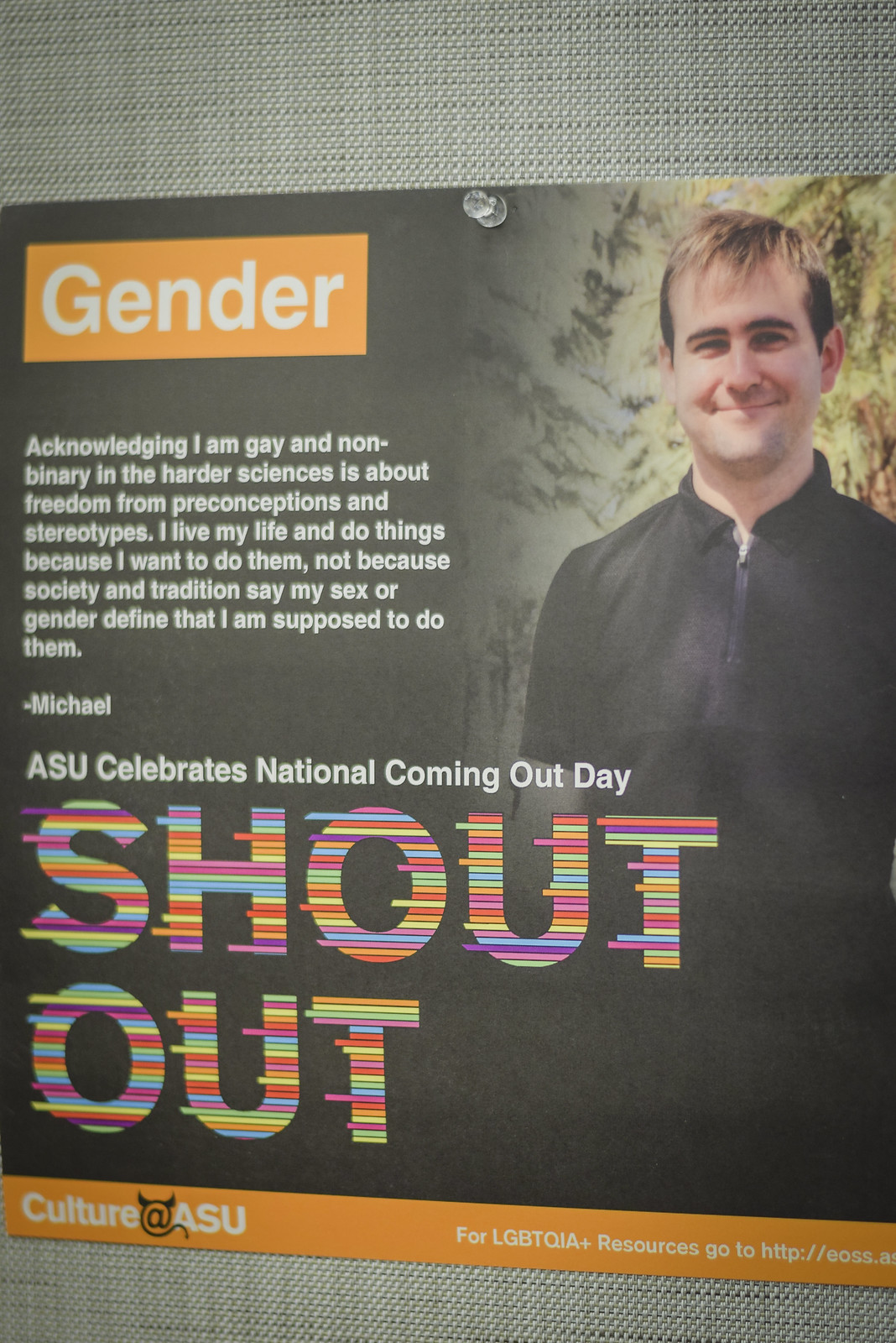The image depicts a flyer measuring approximately six inches high and four inches wide, pinned with a clear pushpin to a gray, woven fabric-covered wall, possibly in a university dorm hallway. The poster is primarily black with distinct graphic elements. In the upper right corner, there is a photograph of a young Caucasian man with blonde hair on top and black hair on the sides, dressed in a black zip-up collared jacket, smiling at the camera. In the upper left corner, an orange text box with white lettering reads "GENDER." Below this box, white text continues: "Acknowledging I am gay and non-binary in the harder sciences is about freedom from preconceptions and stereotypes. I live my life and do things because I want to do them, not because society and tradition say my sex or gender define that I'm supposed to do them." The quote is attributed to Michael. Beneath this, the text announces, "ASU celebrates National Coming Out Day." Midway down the flyer, large, multi-colored letters spell out "SHOUT OUT," with colors alternating in a rainbow-like fashion to evoke a sense of movement. At the bottom of the poster, an orange footer with white text reads, "Culture at ASU." The text continues with a URL for LGBTQIA+ resources, though the website is cut off in the image. This visually striking flyer is likely part of Arizona State University's efforts to celebrate and support National Coming Out Day.